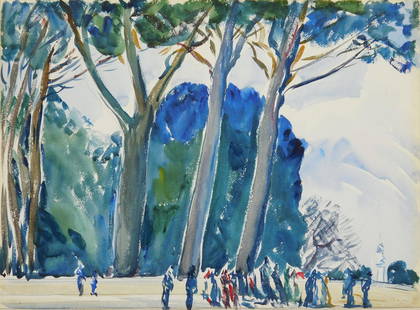The image is a horizontal watercolor painting of an outdoor park setting, characterized by its impressionist style and multiple colors. The foreground features a cream-colored walkway populated by several abstract representations of people, predominantly in blue, teal, and some red hues, moving in various directions. In the lower right corner, there is a group of people and a distinct white statue on a pedestal adjacent to a shrub.

The background on the left side is dominated by a large cluster of three tall trees, with gray and light brown trunks that branch out into green and blue foliage towards the top. On the right side, the sky is depicted with a white, almost undefined watercolor style, suggesting either clouds or clear sky.

The overall scene is bathed in daylight, with the light source coming from the left, casting shadows to the right. Amidst this vibrant park setting, the trees exhibit a mix of lush foliage and bare branches, offering a textured contrast that enhances the depth and serenity of the scene.